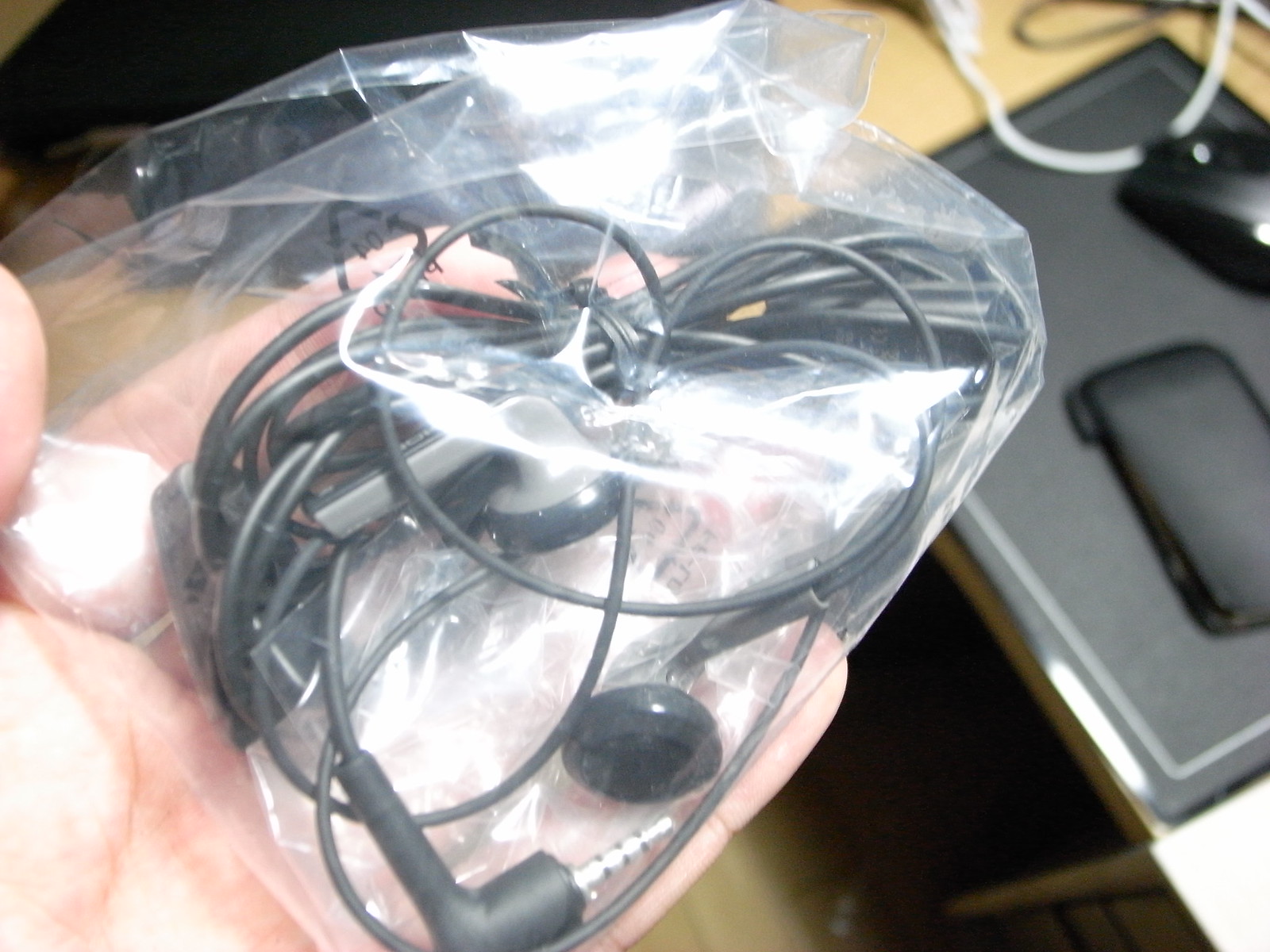This image is an overhead photograph taken indoors, capturing a white male's hand coming from the bottom left, holding a clear plastic baggie with a pair of black wired earbuds inside. The hand is positioned such that the fingertips and part of the palm are visible, with the pointer finger partially seen through the plastic and the pinky hanging off the bottom of the bag. The earbuds are bundled in the middle with a zip tie. In the background, on a brown desk, there is a closed black laptop situated farther away from the bag. On top of the laptop, a black mouse is located in the top right corner along with a black phone placed below it. Additionally, a gray mat and a white Ethernet cord are also visible, adding to the technical equipment spread across the desk's surface. The image does not contain any text and gives an impression of someone organizing or preparing to post the items for sale.